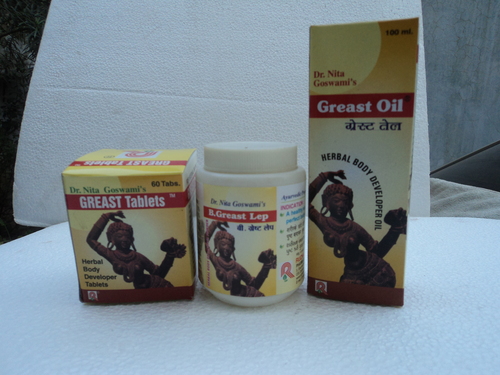On a white surface with a white backdrop, three variations of a product labeled 'GREAST' are displayed, each featuring a distinct form and packaging. The first on the left is a square box labeled ‘GREAST Tablets’. The product in the middle is a cylindrical canister with the label 'GREAST LEP'. The tallest item on the right, a vertically oriented rectangular box, reads ‘GREAST Oil’. Each package is adorned with a detailed image of an orangey-yellow statue of a slender woman. The statue, resembling a hula dancer or a traditional figure, faces the camera while pivoting to the right. Her right arm forms a semi-circle over her head, and her left arm is bent at a 90-degree angle, as if carrying a semi-circular mass. This copper-hued statue serves as a consistent motif across all three products. The largest box also includes the words ‘Herbal Body Developer Oil’ in an arching fashion beside the figure. The packaging predominantly features a yellowish color scheme with red and white text.